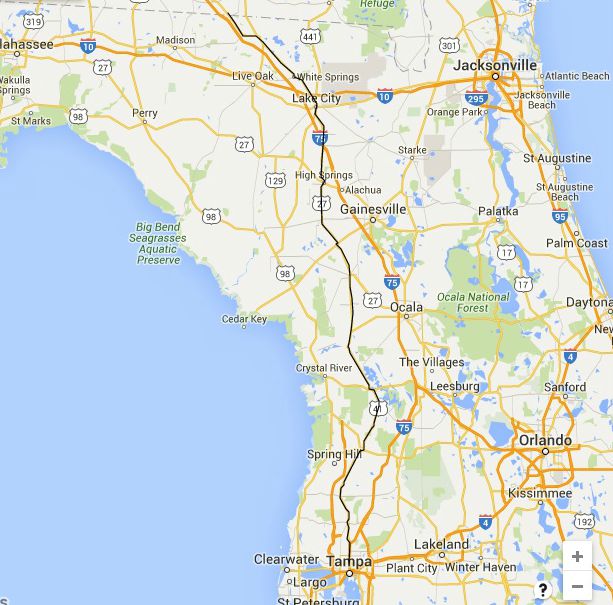The image is a detailed close-up map of Florida, capturing the region from approximately Jacksonville and Tallahassee in the north to Tampa and St. Petersburg in the south. The map prominently features both the Gulf of Mexico on the left side and a portion of the Atlantic Ocean in the upper right-hand corner, depicted in blue. Major cities such as Jacksonville, Tallahassee, Orlando, and Tampa are highlighted with bold black text. The map is intricately detailed, showing a myriad of towns including Gainesville, Lakeland, Clearwater, St. Augustine, Leesburg, and many more. The land is primarily colored yellow, with green areas designating regions like the Ocala National Forest. Various lines in dark and light orange as well as black traverse the map, though their specific designations are not clarified. The map's focus on prominent urban centers and geographical features provides a comprehensive view of this section of Florida.